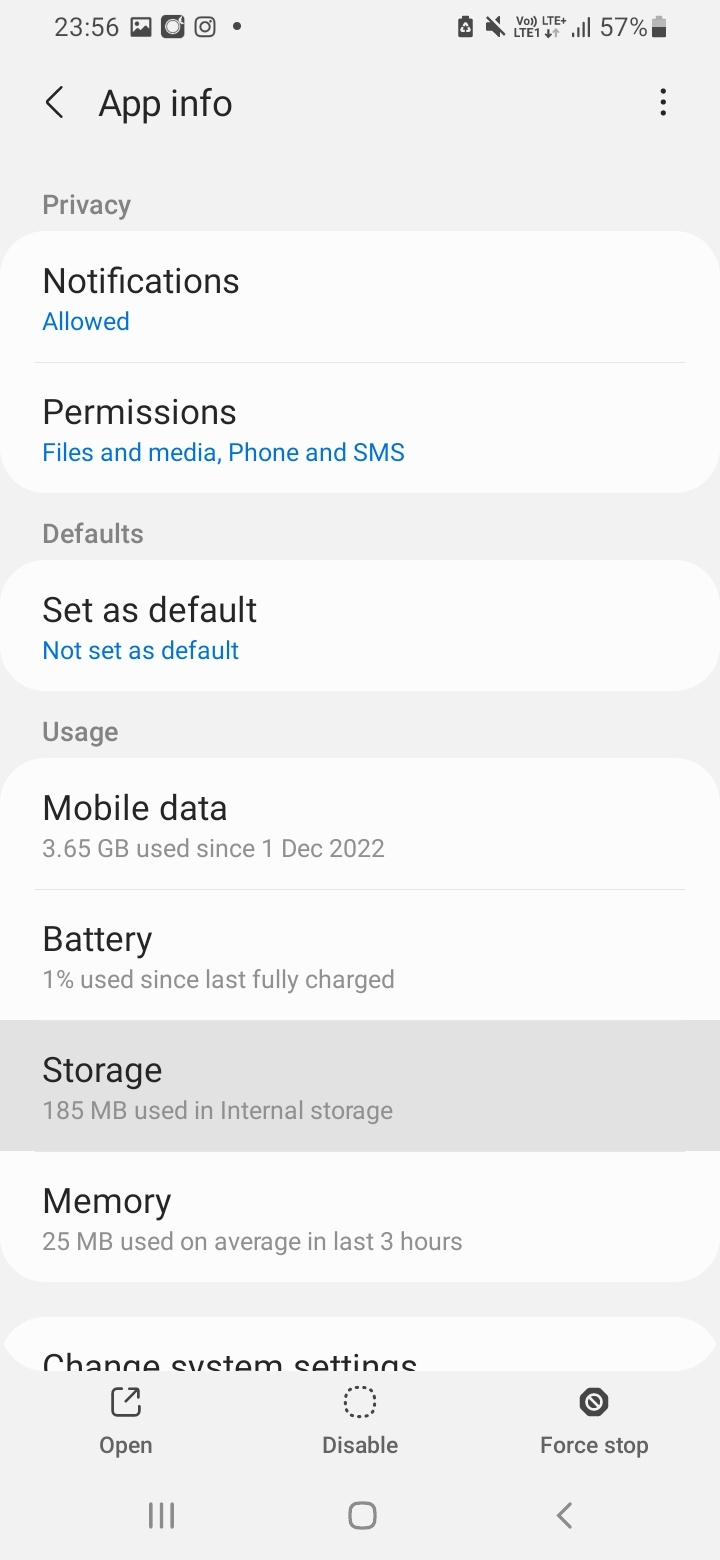This screenshot captures an informational page from a cell phone, detailing comprehensive app data and settings. The background is a clean design using white and light gray hues.

At the top left corner, the time is displayed in black text as "2356," followed by a small picture icon and a camera icon. Below this sequence is a left-pointing directional arrow adjacent to the label "App Info" in black text. To the right, a muted speaker icon precedes the network information which shows "LTE," the connectivity bars, a "57%" indicator, and a battery icon.

Further down, three vertical black dots signify additional menu options. To the left, the first section lists "Privacy," followed by "Notifications," with the status "Allowed" highlighted in blue text beneath it. Next is the "Permissions" section in black text, with specifics like "Files and Media," "Phone," and "SMS" delineated in blue text.

Continuing, the "Defaults" section includes the option "Set as Default," marked with blue text as "Not Set as Default." Then, an "Usage" section indicates 3.65 gigabytes of mobile data used since December 1, 2022, while the "Battery" section shows 1% usage since the last full charge. The "Storage" section notes 185 megabytes used in internal storage, and the "Memory" section averages 25 megabytes used over the last three hours.

At the bottom, options for "Open," "Disable," and "Force Stop" allow user interactions with the app.